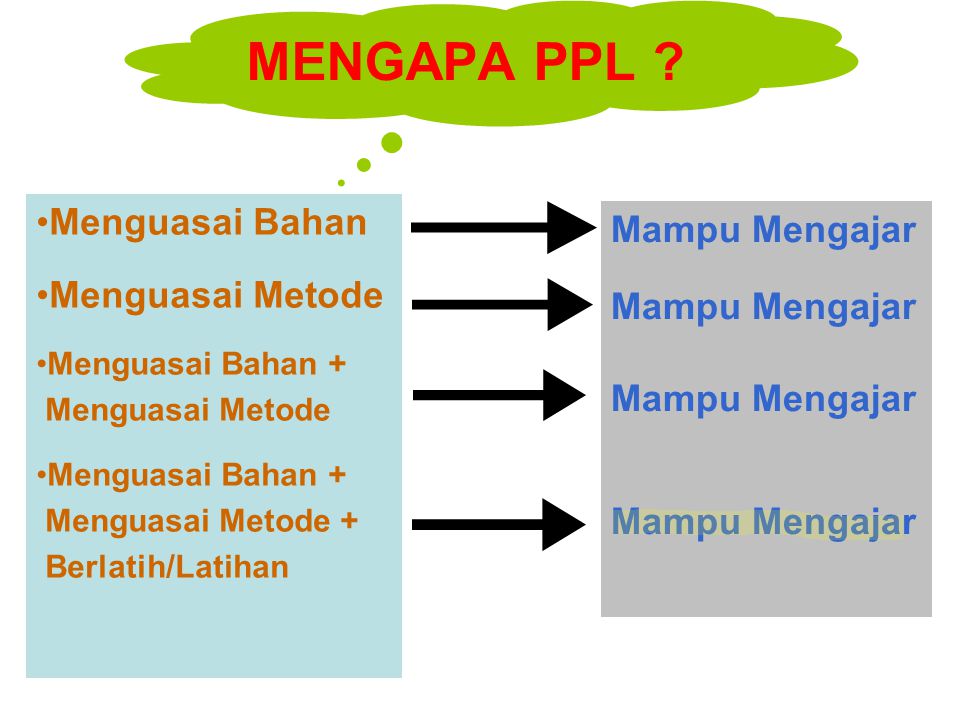This image appears to be a slide from a PowerPoint presentation featuring a tri-colored themed layout. At the top, there's a green cloud-like speech bubble containing red text which reads "MENGAPA PPL?" Next, underneath this green bubble, a large light blue rectangular box occupies the left side. The blue box includes an orange bullet-pointed list that states: "MENGU-ASAI-BAHAN," "MENGU-ASAI-METODE," "MENGU-ASAI-BAHAN-PLUS," "MENGU-ASAI-METODE-PLUS," and "BARLANI/LATAHAN." Four arrows in black point rightward from this blue box to a light gray rectangular box on the right side. Inside the gray box, blue text is repeated four times: "MAMPU MENGAJAR." The last "MENGAJAR" is subtly highlighted with a faint yellow marker. The slide appears to be structured, possibly for educational or business purposes.